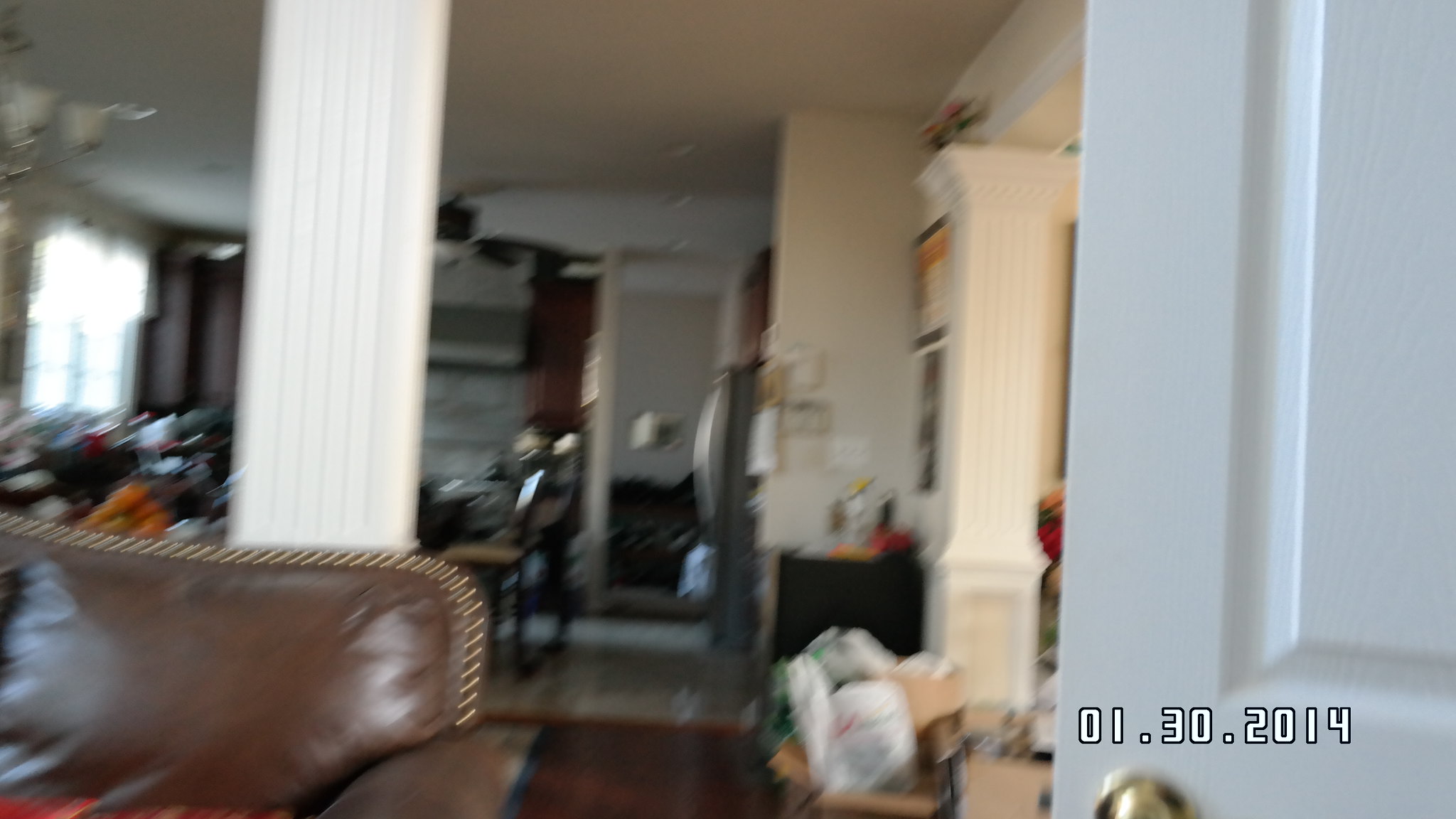A blurry, indoor photograph with a rectangular frame dated "01.30.2014" in white text at the bottom right corner. On the right side of the image, an open white door is visible, with a golden-colored doorknob at the bottom. The white ceiling forms the upper section of the image. In the bottom left corner, there is a dark brown chair or couch, partially blocking view of a white pillar directly behind it. Further in the background, another chair can be seen, adding depth to the scene.